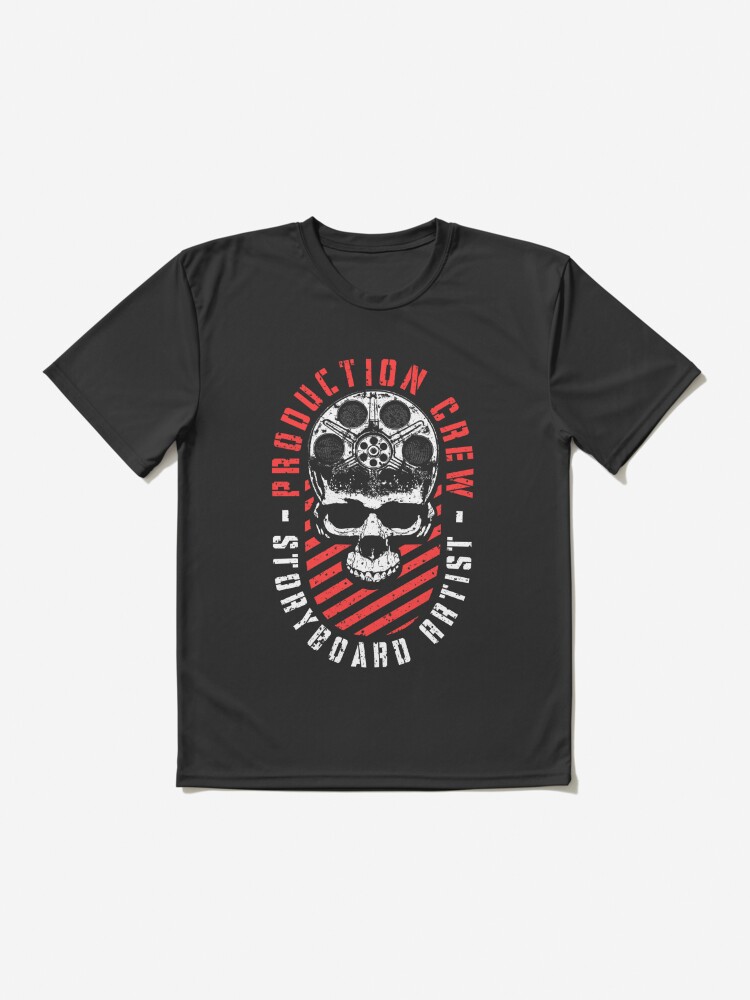The image features a black short-sleeved t-shirt made of cotton, spread out on a light grayish or plain white background. The central design on the shirt prominently displays a white skull with a movie reel integrated into the top of the skull. Surrounding the skull in an oval outline is the text "Production Crew" in red at the top and "Story Board Artist" in white at the bottom. Below the skull, there are diagonal red stripes. The shirt has a casual look, reminiscent of a band t-shirt, with no other text or design elements besides the mentioned phrases and skull graphic.